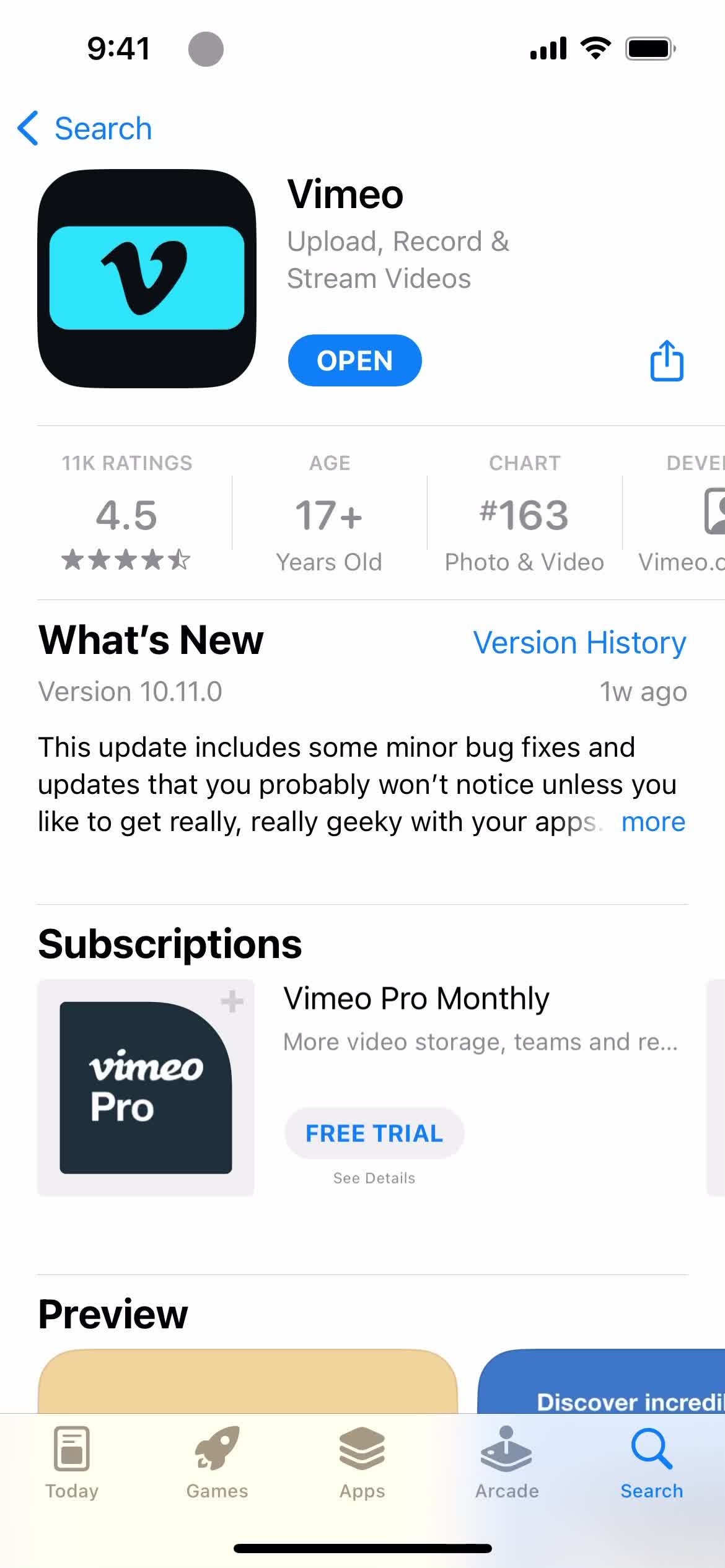Here is the cleaned-up and detailed descriptive caption for the image:

---

At the top of the cell phone screen, the status bar displays "9:41" on the left, followed by a gray circle. On the right side, signal bars indicate cellular service, alongside icons for Wi-Fi and a fully charged battery.

Just below the status bar, on the left side, there is a green arrow icon next to the word "Search" in green text. 

Beneath this, a black box encompasses a black and turquoise rectangle, which contains a black 'V'.

To the right of this box, text reads: "Vimeo: Upload, record, and stream videos," followed by a blue button labeled "Open" in white text.

An additional icon featuring a box with an upward-pointing arrow is located further to the right. 

A light gray line separates this section from the information below.

Starting from the left, the next section states: "11,000 ratings" accompanied by "4.5 stars", and "Age 17+ years old." Further right, it reads "Chart: #616 in Photo & Video."

Below, the "What's New" section highlights the update details: "Version 10.11.0" is specified, with "Version History" as an active blue link to the right. The update, released one week ago, includes minor bug fixes and updates that may go unnoticed unless scrutinized by tech enthusiasts. Text fades out and concludes with "more" in blue.

Following another gray divider, the "Subscriptions" section presents information: "Vimeo Pro" and "Vimeo Pro monthly - more video storage, teams..." next to a gray button with the text "Free trial" in blue. Below this is a gray "See details" link.

A final gray line precedes the "Preview" section.

---

This caption provides a clear and organized summary of the various elements and sections visible on the cell phone screen.